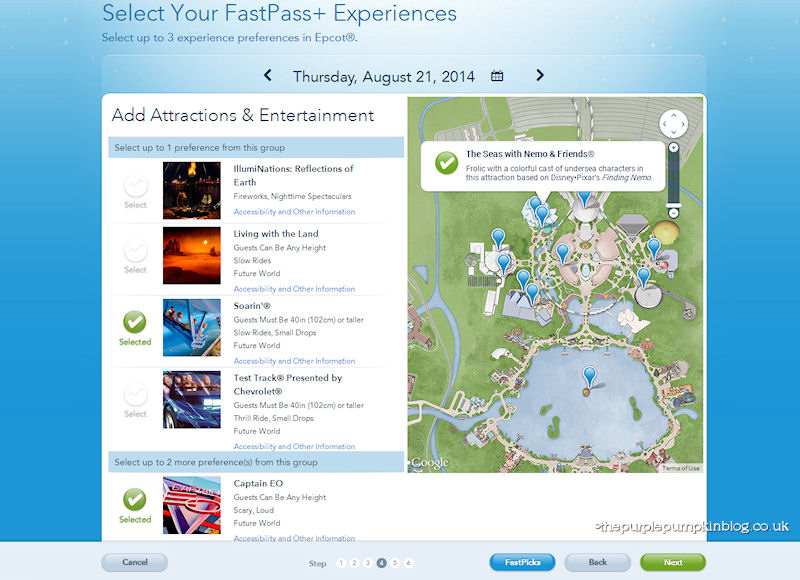The image appears to be a screenshot from a computer interface for selecting FastPass+ experiences at Epcot. The background is primarily blue, with the main focal point being a white screen in the middle. At the top of this screen, in blue text, it reads “Select Your FastPass+ Experiences.” Additional text instructs users to “select up to three experiences," emphasizing preferences in Epcot, and mentions the date, Thursday, October 21st, 2014.

On the right side of the screen, there is a map likely showcasing the layout of the park. A white popup with a checkmark next to it indicates that "The Seas with Nemo and Friends" has been selected. To the left of the map, there is a list of attraction choices that the user is scrolling through. Among the checked attractions are "Soarin'" with a note that guests must be 40 inches or taller, featuring descriptors like slow rides, small dogs, small drops, and Future World. Another selection is "Captain EO," which highlights that guests can be any height and includes descriptors such as scary, loud, and Future World.

At the bottom of the interface, there are several navigation buttons: a gray Cancel button, a blue "Fast Picks" button, a gray Back button, and a green "Next" button.